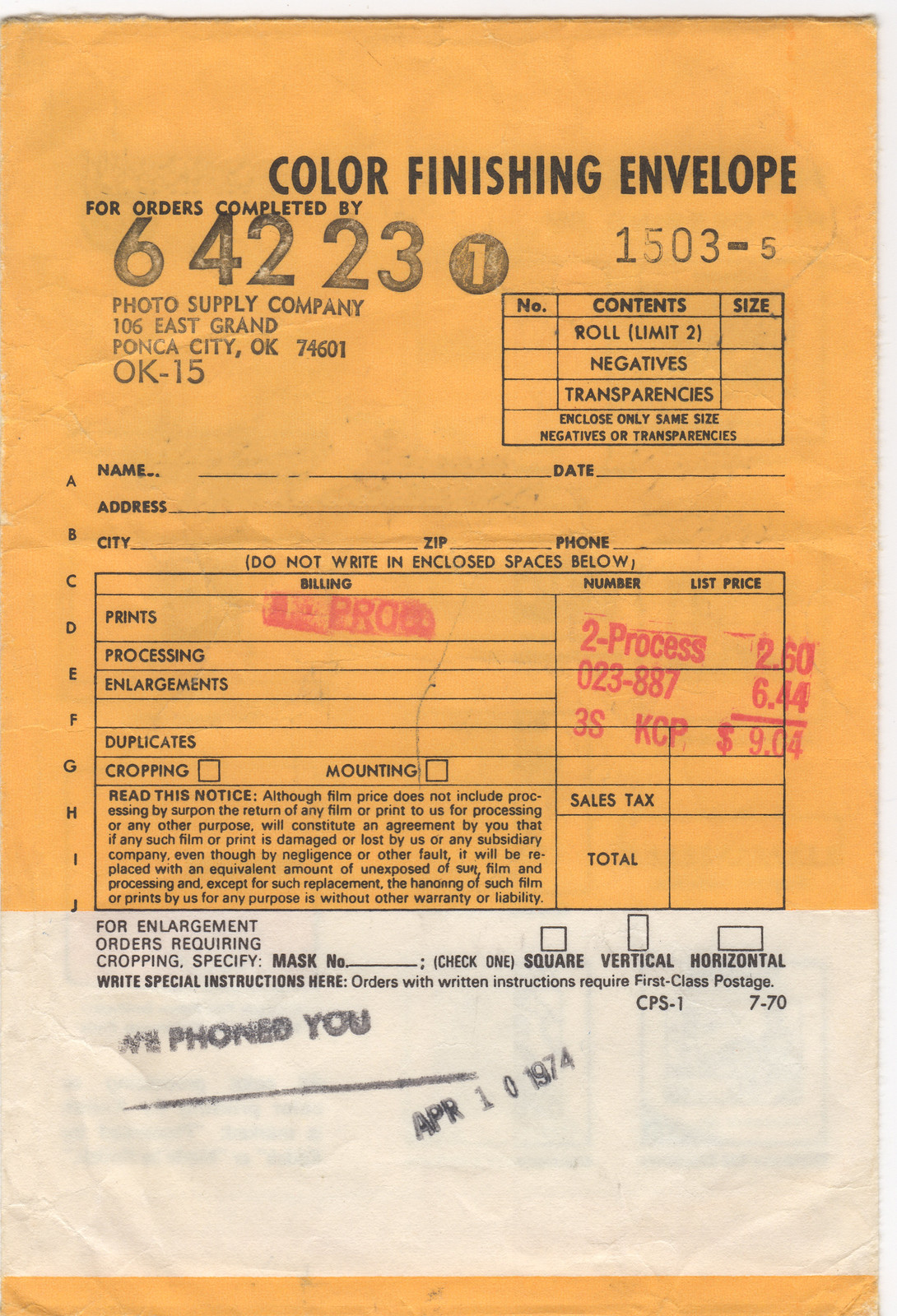The image depicts a vintage manila orange-colored envelope labeled as a "Color Finishing Envelope" from a photo supply company. The top section of the envelope features the text "Color Finishing Envelope" in black lettering. Below this, it's noted for orders completed by a stamp number "642-31" along with an additional number "1503". On the right-hand side, the address is listed as "Photo Supply Company, 106 East Grand Street, Ponca City, Oklahoma 74601". The envelope includes multiple sections for filling out details such as the recipient's name, date, address, city, zip code, and phone number, along with checkboxes and spaces to specify the type of prints, processing instructions, enlargements, duplicates, cropping, and mounting requirements.

Further details include a disclaimer about film pricing, and there are red stamps indicating costs, with descriptions such as "$62.60" and "$6.44". The bottom section, which is white, includes a note stating they contacted the recipient on "April 1st, 1974" and directions for enlargement orders requiring cropping. There are also spaces for specifying preferences like roll limits, negative and transparency handling – highlighting that only same-size negatives or transparencies are included. The overall impression is that this is an old Kodak shipping or processing envelope used for photo development purposes.